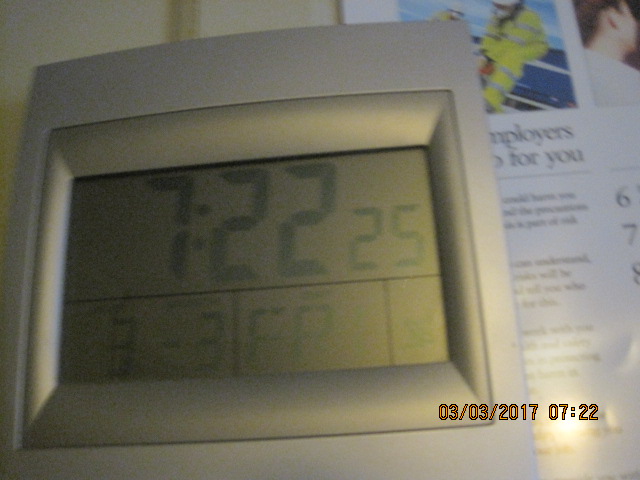The image features a close-up of an alarm clock set against a silver metallic base. The clock itself has a gold outer casing and a gold face, with black digital numerals displaying the time as 07:22. Below the time, the date is indicated as 03-03. The clock screen appears to be covered with glass, with some blurred text at the bottom that may read "FP," though it is not clearly legible.

In the background of the image, there are several papers. One piece of paper mentions "employers" in black text and features a picture of an individual in a yellow uniform with silver stripes, wearing a white helmet. Another paper to the right shows part of a person's head with dark hair, who appears to be Caucasian, and is wearing a white shirt. This paper also has the numbers "67," but the text is mostly unreadable.

The background features a beige wall. The image has a date stamp of 03-03-2017 at 07:22, which corresponds with the time displayed on the clock.